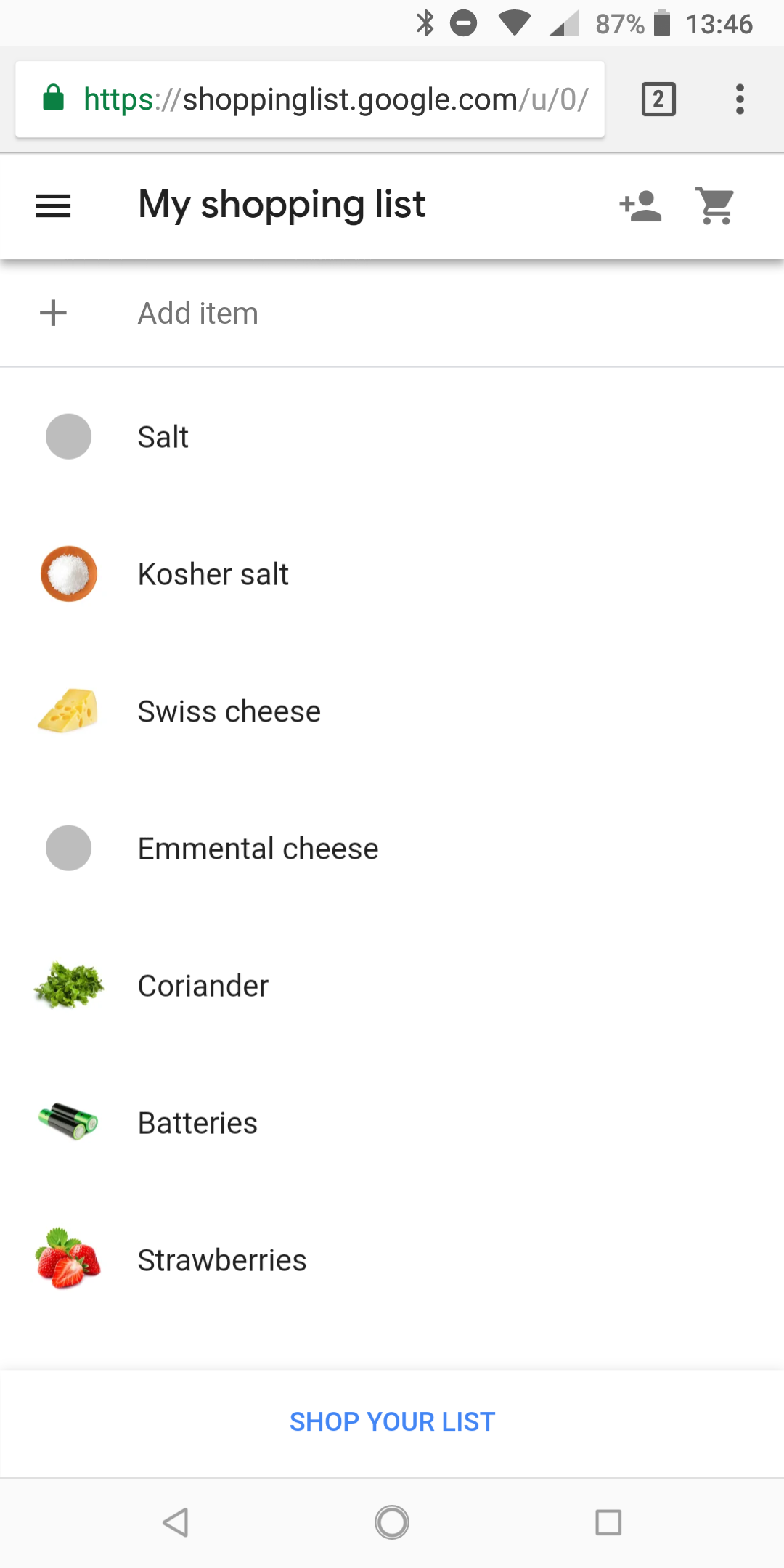The screenshot depicts a smartphone screen with a predominantly white background. In the upper right corner, the time is displayed as 13:46 next to a battery icon showing an 87% charge. The wireless connection icon indicates a weak signal, as only one bar is filled. Adjacent to these icons, a secure green padlock accompanies the web address, "shoppinglist.google.com/u/0", indicating a secure connection.

The main header reads "My Shopping List" against the white background. Below this header, a "+" sign next to "Add Item" allows the addition of new list items. The shopping list displays various items, each accompanied by simple line drawings. The listed items include: salt, kosher salt, Swiss cheese, Emmental cheese, coriander, batteries, and strawberries.

At the bottom center of the screen, in blue capital letters, the text "SHOP YOUR LIST" is prominently featured. Finally, at the very bottom of the screen, there are three light gray navigation icons: a circle in the center, a square on the right, and a triangle pointing to the left on the left side.